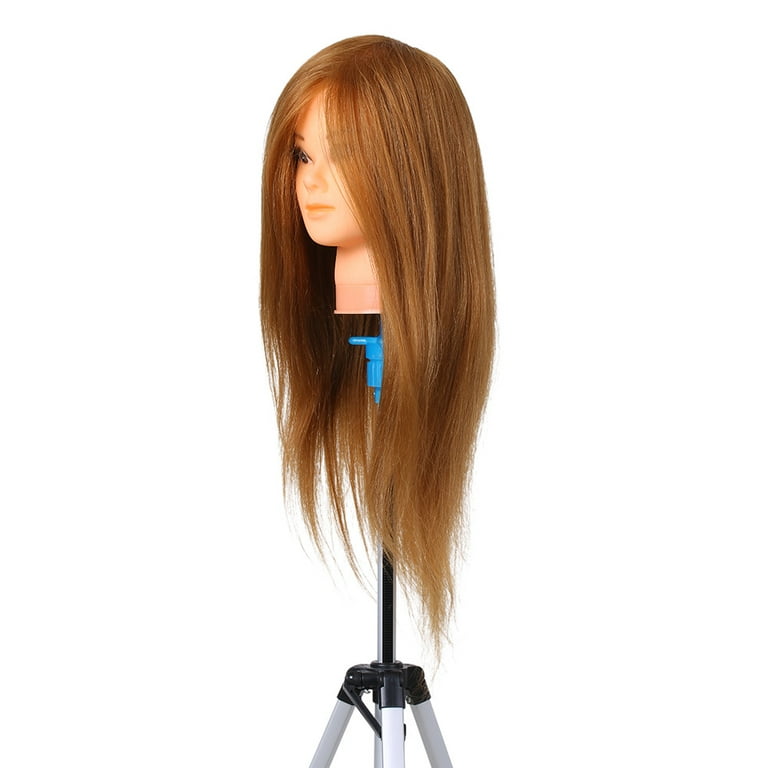The image showcases a mannequin head mounted on a blue-topped, adjustable tripod. The mannequin, featuring a young female face with two eyes, a nose, mouth, and eyebrows, is oriented to the left against a plain white background. Its wig, which is long, brownish-red with golden and honey highlights, looks freshly brushed and cascades straight down both sides of the face, parted neatly in the middle. The hair ends are somewhat uneven and shaggy, hinting it might be used by a trainee hairdresser for practice. The mannequin's white head and neck are clearly visible, supported by the tripod, of which only the blue top and part of the skinny pole are in view. The overall focus is on the mannequin's detailed facial features and the rich, finely textured hair.